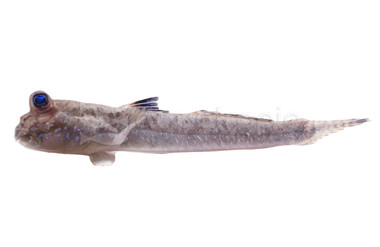This photograph features a small, slender fish, positioned against a white background and facing left. The fish's most striking feature is its large, bright blue eyes, which are situated more on top of the head rather than on the sides, giving it a somewhat cartoonish appearance. Its body is predominantly a pale beige color adorned with dark polka dots, while lighter blue or violet spots are scattered along its underside, perhaps to confuse predators by reflecting sunlight. This fish also has a stubbed nose and a very small mouth with thin lips. Its fins include a notably dark, almost black dorsal fin, blue top fins, and a semi-transparent, pointed tail fin. The unusual eye placement and the overall color pattern give the fish a unique and almost whimsical appearance.